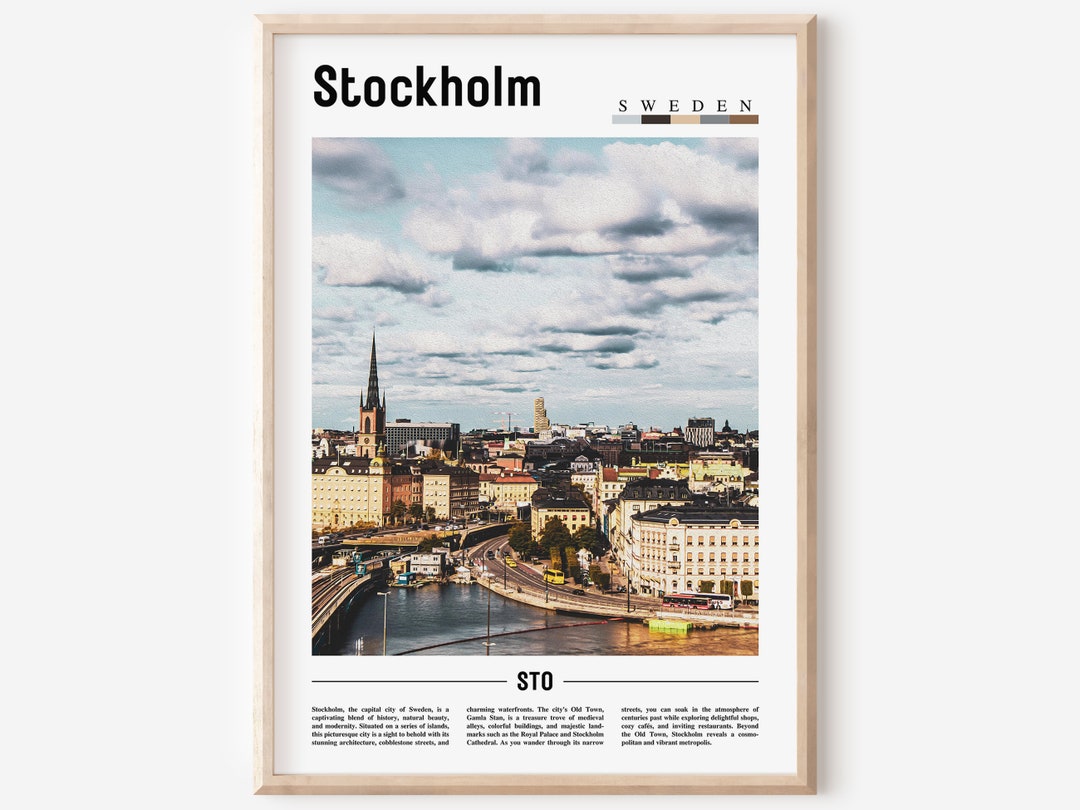This framed poster, set against a neutral white wall, beautifully showcases the cityscape of Stockholm, Sweden. The frame is a light tan color, and the poster itself has a white background. At the top left, "Stockholm" is prominently written in large black letters, while "Sweden" appears to the top right in smaller black font, underlined by a sequence of colored blocks in gray, black, cream, tan, and brown. Below these texts, an aerial view of the city is displayed, revealing a stunning cityscape with a body of water in the middle. On one side of the water, there are railroads, and on the other, a freeway or two-lane road lined with streets and numerous buildings, including a tall church steeple. The skyline features beautiful, seemingly French Revolutionary-style buildings made of concrete or stone with black roofs and numerous windows. The sky above is a big, blue expanse with a slightly cold hue. At the bottom of the image, the letters "STO" are prominently displayed between two horizontal lines, followed by three paragraphs of text that presumably describe the city. The overall presentation suggests a stylish blend of historical and modern elements, encapsulated in a detailed and picturesque format.